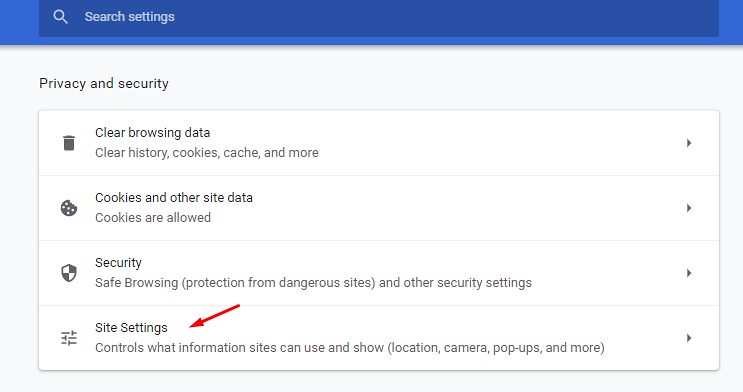A detailed informational screenshot provides a comprehensive view of various privacy and security settings. At the top of the image, a blue rectangular header contains a magnifying glass icon next to the words "Search settings" in white text. Below this header, the background turns white, featuring black text that reads "Privacy and security."

Under this heading, there are four distinct options presented within a white rectangular box. The first option is "Clear browsing data," accompanied by a dark gray garbage can icon. This section seems interactive, indicated by a right-facing arrow on its far right side.

The second option is labeled "Cookies and other site data," featuring a dark gray icon of a cookie with bites taken out of it. It indicates that cookies are currently allowed.

The third section includes a white and dark gray checkered shield icon, labeled "Security." This option provides details on safe browsing, including protection from dangerous sites and other security settings.

The last option, highlighted with a red arrow overlay to emphasize its selection, is titled "Site settings." This section controls what information websites can access and display, such as location, camera, pop-ups, and more.